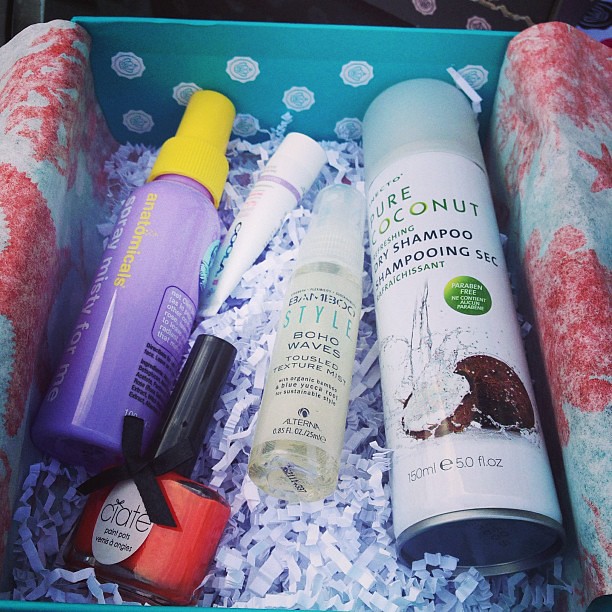The image depicts a festive gift box in a teal shade adorned with white polka dots and filled with various health and beauty products. The box, brimming with blue and salmon-colored tissue paper and white crinkle paper, contains an assortment of items placed on a bed of shredded white paper. Among the products are a white can of pure coconut dry shampoo featuring a pale blue lid and a picture of a coconut, and a purple bottle of bamboo style boho wave texture mist with a yellow cap. There's also a clear bottle with a greenish tint, a white can of spray, and a coral-colored nail polish with a black lid. The thoughtful presentation suggests it is intended as a thank-you gift.